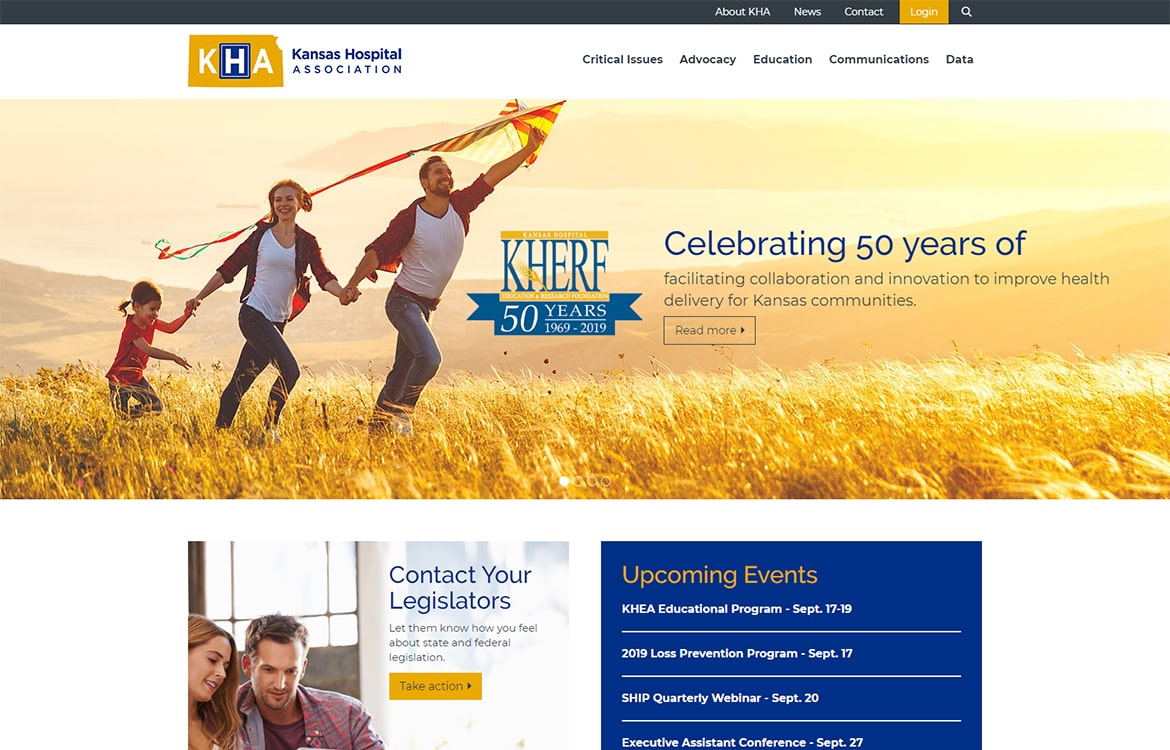A detailed screenshot of the Kansas Hospital Association (KHA) homepage is displayed. The header bar is gray, featuring navigational links to "About KHA," "News," and "Contact" on the right, with a yellow login button and a magnifying glass search icon. Occupying the top section is a background photograph of a picturesque golden field, showing a man, woman, and girl joyously running, with the man holding a kite. 

Overlaying the photograph is the KHA logo, an attractive blend of blue, white, and yellow. Adjacent to the logo is the emblem for KHERF, accompanied by a big blue text proclaiming "Celebrating 50 Years Of." Beneath this, a tagline reads, "Facilitating Collaboration and Innovation to Improve Health Delivery for Kansas Communities," with a small yellow "Read More" button underneath.

The bottom section of the screenshot transitions to a white background. On the left, a photograph portrays a man and woman examining something together, with text beside it encouraging visitors to "Contact Your Legislators," highlighted by a yellow "Take Action" button. To the right is a dark blue box listing upcoming events, such as the KHEA Educational Program, 2019 Loss Prevention Program, SHIP Quarterly Webinar, and Executive Assistant Conference. The bottom of the image lacks a border, giving a clean and continuous appearance to the layout.